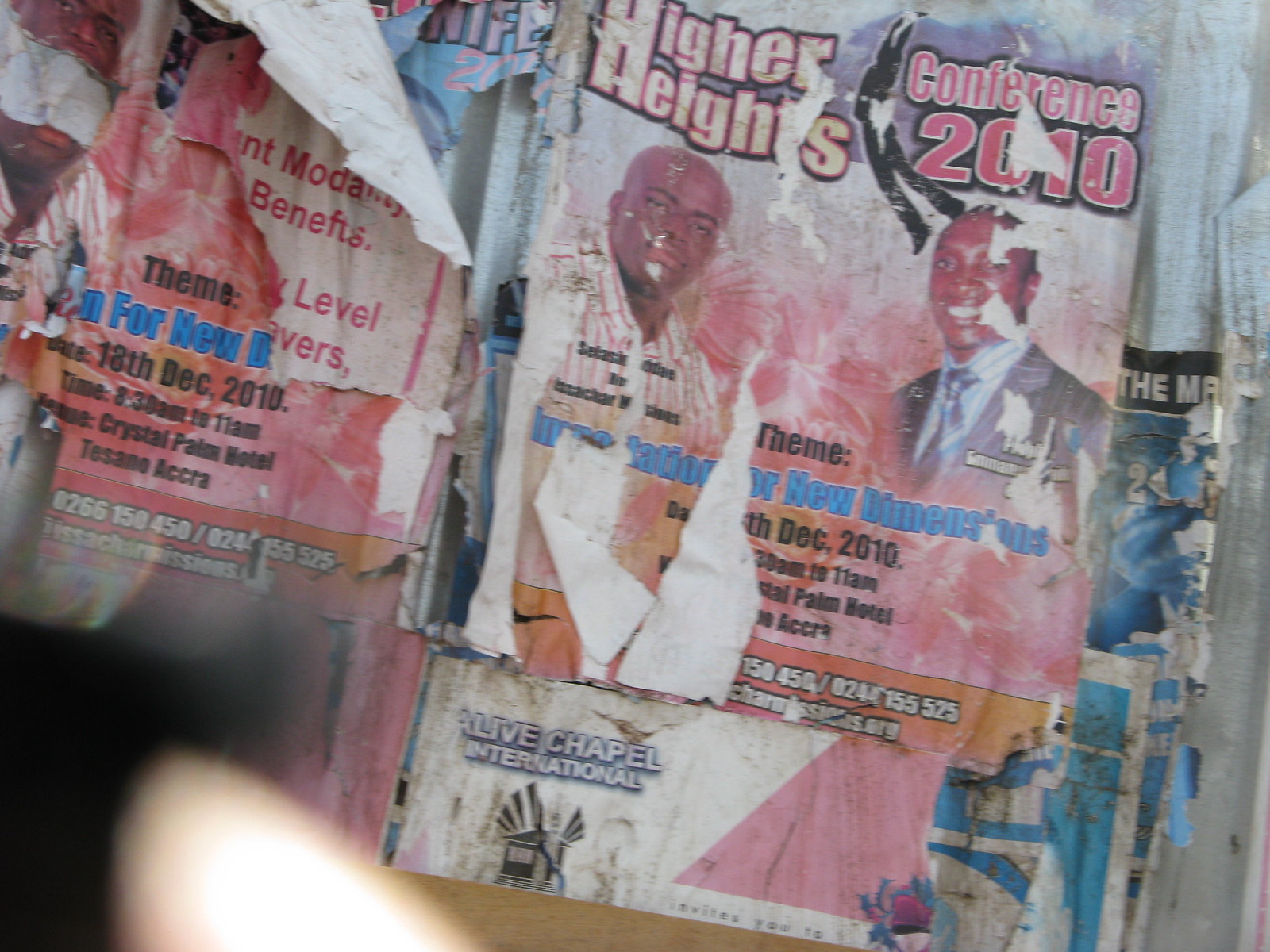The large square image depicts a weathered stone wall plastered with layers of deteriorated posters. The most prominent poster, located towards the upper right, advertises the "Higher Heights Conference 2010." It features two Black men; the man on the left is bald, wearing a white and pink striped shirt, while the man on the right, also bald, is dressed in a blue pinstripe suit with a white collared shirt and blue tie. Both men face the camera and smile. The poster contains fragmented text, including "theme: New Dimensions" and "December 10, Palm Hotels," though much of it is unreadable due to rips and wear. Surrounding this main poster are various other degraded flyers, showcasing an environment where new posters are frequently layered over old ones without removing them. The entire scene suggests an outdoor setting, evidenced by the weathered appearance of the posters. In the lower left-hand corner of the image, a blurry spot appears to be the finger of the person taking the picture.